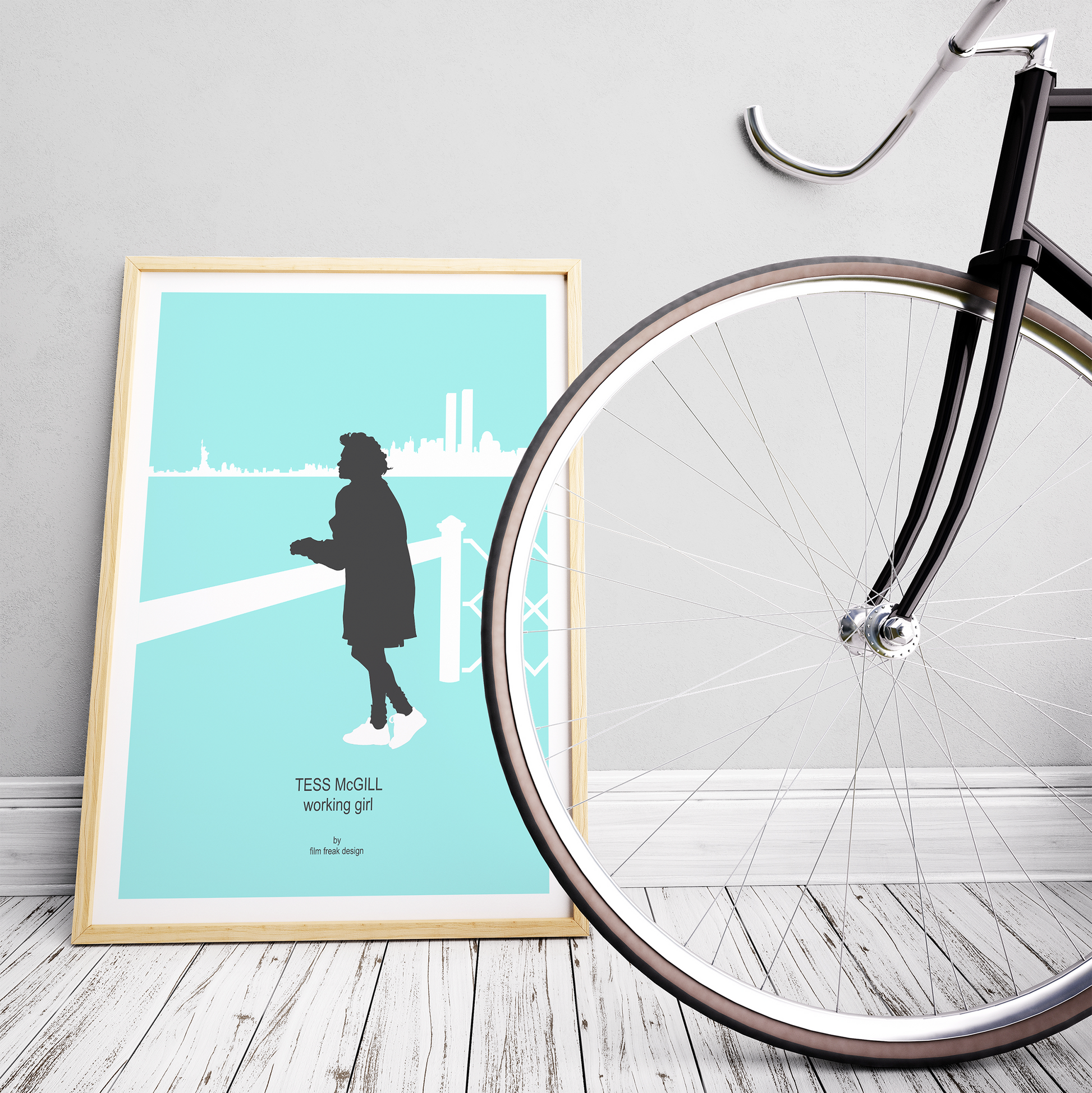The photo captures a scene with a prominently displayed bicycle wheel on the right side. The bike has thin metal spokes and a black frame, with a sleek silver handlebar. Resting on a hardwood floor, painted white but still revealing the wood grain, the wheel appears vintage. Adjacent to the bicycle, on the left side of the frame, hangs a light brown-framed artwork. This artwork features the silhouette of a woman, in black, wearing white shoes, leaning on a bridge with the backdrop of New York City. The city's skyline, including the Statue of Liberty and skyscrapers, is rendered in white against a light green or sea-blue background. The image includes text that reads "Tess McGill, Working Girl," though the smaller text is illegible. The setting appears to be indoors, with the scene positioned against a gray wall.